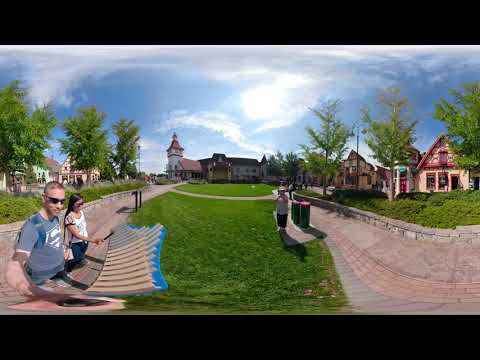In this vibrant panoramic image, a young couple, seemingly tourists, are seen walking through a picturesque town square under a bright blue sky adorned with wispy white clouds and a bright, round sun partially veiled by clouds. The man, wearing sunglasses and a blue Superman t-shirt, leads slightly ahead of the woman, who has long dark hair, shades, a light top, and dark pants. They are positioned towards the left side of the image, standing near a tan wooden stick board against a blue background. Around them, the town square unfolds with freshly cut grass separating two brown stone sidewalks. The scene is framed by idyllic homes with peaked roofs and occasional tall towers stretching across the horizon, accompanied by verdant trees. Another individual, also appearing as a tourist, is seen near a stretch of green lawn and a row of wooden planks on the right side, close to a brick and concrete path. The entire setting suggests a serene European village, possibly in the Netherlands, with beautifully maintained buildings basking in the sunlight.